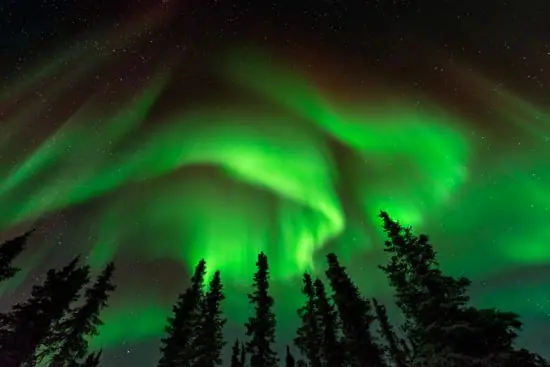This color photograph captures the mesmerizing Aurora Borealis, or Northern Lights, illuminating the night sky with an ethereal display of luminescent green hues. Taken from a low angle, the camera points upwards, silhouetting the tops of tall, spindly pine trees typical of cold northern climates against the vibrant sky. The sky is bathed in a brilliant lime green, with various shades swirling across the expanse. At the center, the light intensifies to an almost white brilliance, accentuating the swirling patterns. The upper part of the image remains dark, providing a striking contrast to the luminous green waves that traverse the sky. The photograph also features faint white spots resembling stars, enhancing the surreal beauty of this natural phenomenon. Despite the photograph's slight blur and pixelation, it vividly conveys the awe-inspiring spectacle of the Northern Lights dancing above a serene forest.